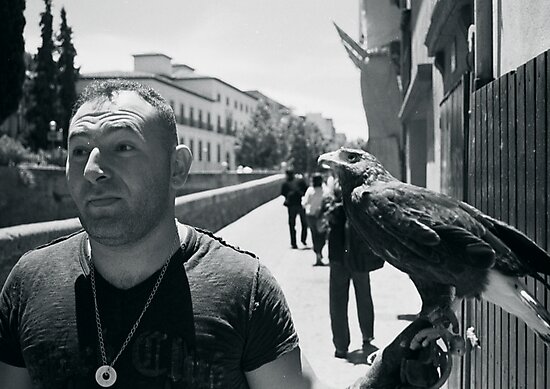In this black-and-white photograph, a man, possibly in his late 20s or early 30s, stands slightly to the left of center. He has short hair and is wearing a dark-colored t-shirt, though the exact details of the shirt are unclear due to the grayscale nature of the image. Around his neck hangs a circular necklace with a medallion. The man is not looking at the camera and appears to be holding a bird, possibly a hawk or raven, on his left hand, which is protected by a glove. The bird is primarily brown with a lighter underbelly and is gazing intently at the man.

In the background, partially obscured, are several people standing on what seems to be a walkway. To the left of the man, a low stone wall and a large building or house can be seen, with some trees adding to the scene. On the right, a wooden fence or gate is visible, emphasizing the public and possibly urban environment of the photograph. The overall setting appears to be outdoors on a sunny day, and the image does not have the polished look of a professional shot, giving it a candid and spontaneous feel.